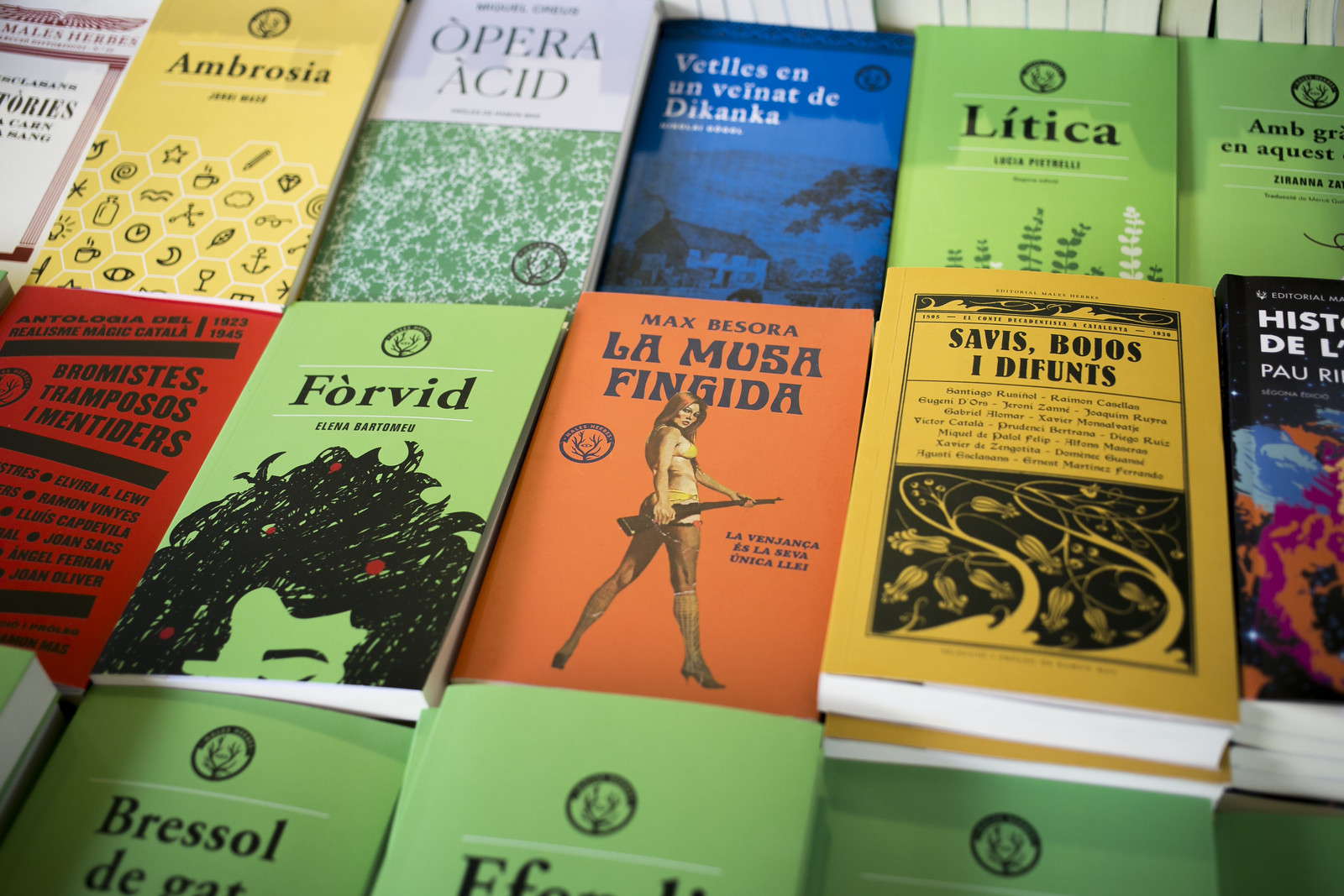This photograph features a collage of book covers, neatly spread out in three slightly diagonal rows across a table. The books are all of similar size, although the scale is not clearly discernible. Many of the covers are in various shades of light blue, creating a visual pattern. Prominently, there is an orange book with dark purple lettering in the middle. The cover depicts a woman with red hair clad in a yellow bikini and heels, holding a rifle, and looking back at the camera.

The top row includes titles such as "Ambrosia," "Opera," "Acid," "Vettels in Un Vecnak de Dikanka," and an unreadable one, all seemingly in foreign languages. The middle row features titles like "Dramistes," "Tramposos," "Mintinders," "Forvid," "La Musa Fingida," "Sabes," "Bojos y Difunts." A red book with black writing, partially unreadable, sits alongside the others. Finally, the bottom row consists of green books in varying shades, with their titles mostly obscured or cut off, making them difficult to read. The vibrant colors and different languages showcased on the covers suggest a diverse and eclectic collection.